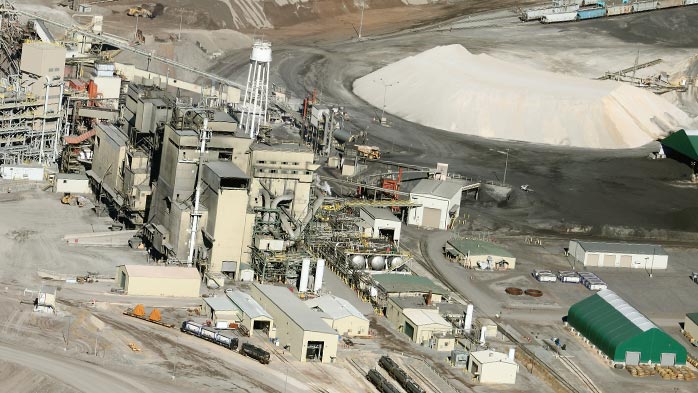The aerial shot depicts an expansive industrial area, likely a rock quarry or mining facility. The left side is densely packed with large white industrial buildings, including garages, sheds, and a small white water tower. In contrast, the right side features a massive mound of light-colored sand or gravel, almost as tall as the buildings themselves, surrounded by dark, asphalt-like ground. Scattered throughout the image are railcars, particularly in the upper right, suggesting a strong reliance on railroad transport for local industry. Additionally, a green hangar is visible on the lower right, further emphasizing the site's industrial nature. No people are visible in the image, underscoring the focus on machinery and infrastructure in this bustling industrial environment.